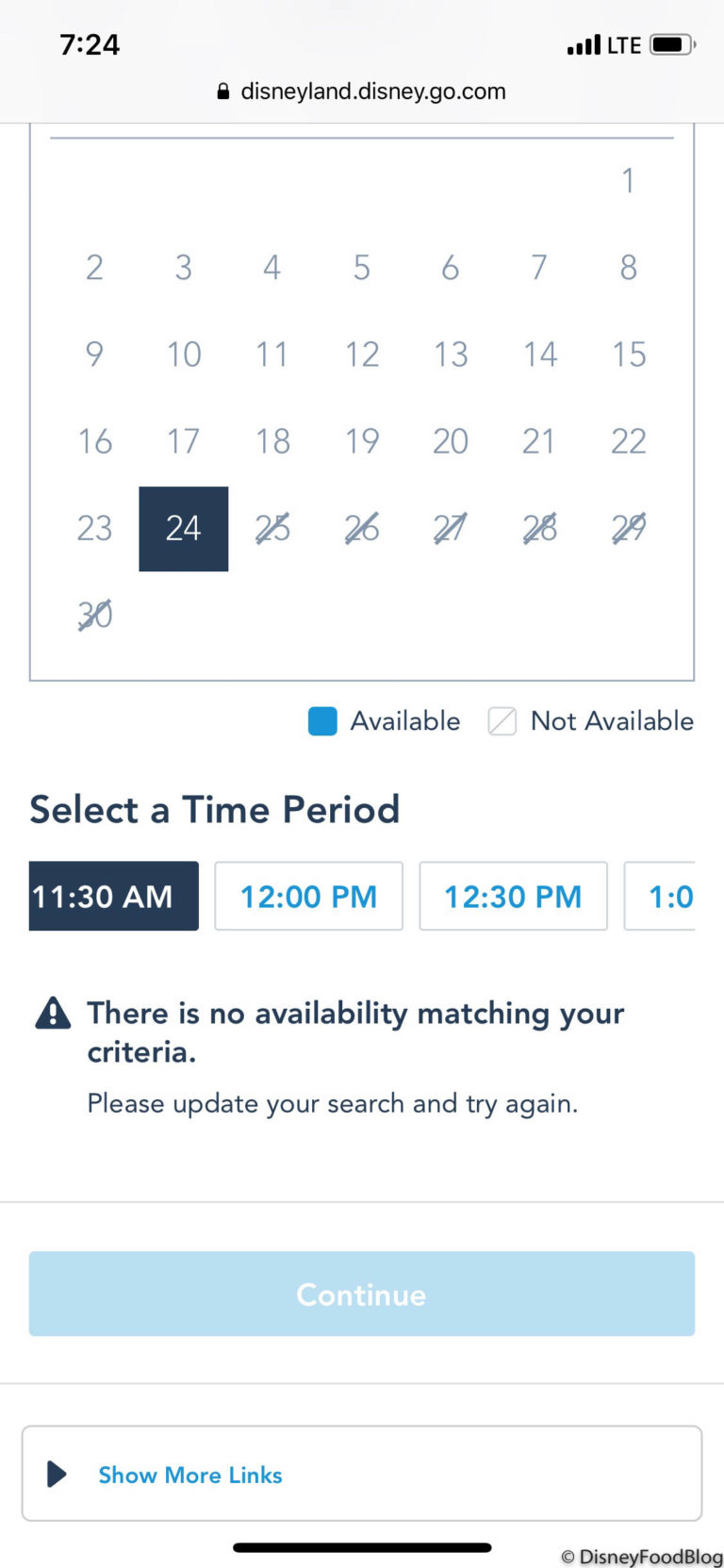The image depicts a mobile interface for purchasing tickets to Disneyland Park. At the top left corner, the screen displays the current time as 7:24 AM, followed by icons indicating the device's connection to Southwest, LTE signal strength bars, and the battery level. 

Below this, the interface features a calendar ranging from the 1st to the 24th, while dates from the 25th to the 30th are crossed out, signifying unavailability. A blue label captioned 'Available' is also crossed out, indicating that no tickets are available for the selected dates.

Further down, the user is prompted to select a time period with options listed as 11:30 AM, 12:00 PM, and 12:30 PM. A message beneath this selection box states, "There is no availability matching your criteria. Please update your search and try again." Below this message, a horizontal line is followed by a blue rectangle button labeled 'Continue.' 

At the very bottom, the screen features a text link reading 'Show more links' and a black line that leads to the 'Disney Food Blog.' The entire visual suggests that it is an interface for purchasing Disneyland Park tickets, highlighting the lack of available slots for the chosen dates and times.